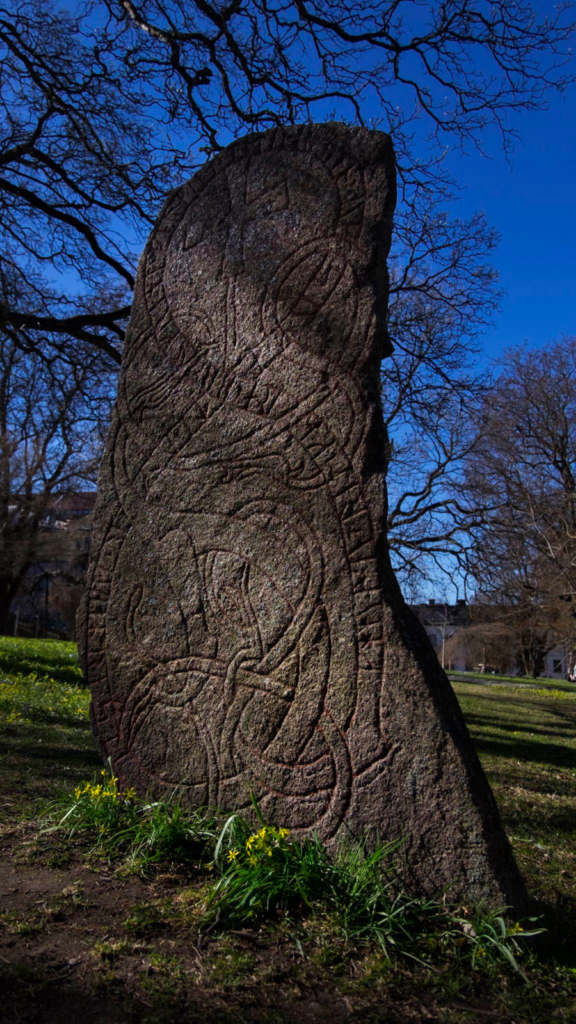The image showcases a serene outdoor scene under a bright blue sky, featuring a central focal point of a tall, thin stone statue with intricate engravings. This dark brown, possibly ancient stone is adorned with geometric patterns, swirling motifs, and a prominent cross inscribed at the top, lending it an air of historical significance. The stone stands amidst a lush field, with patches of dark green grass and sprouting yellow flowers at its base, contrasting against the surrounding brown dirt. Flanking the stone, sparse trees—some tinged black and scant of leaves—reveal more of the vivid blue sky, adding depth to the composition. To the right and left, low-rise brown buildings with brown roofs, alongside slightly taller silhouettes, punctuate the horizon, blending seamlessly with the landscape.